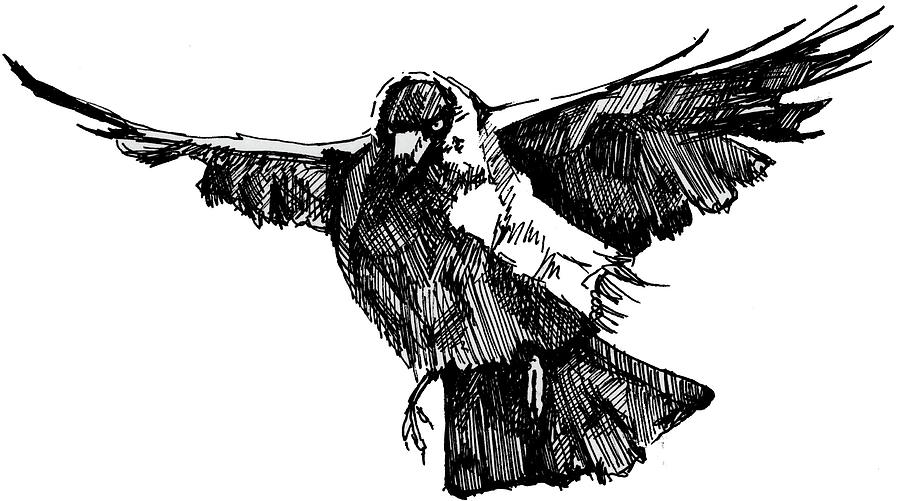This image is a detailed black and white etching of a crow in flight, rendered in an expressive scribble style using black ink on a white background. The crow is prominently positioned at the center of the frame, its wings outstretched in a large arc, demonstrating a sense of dynamic movement. The bird's eyes appear fierce and menacing as it stares directly at the viewer, creating an intense focal point. Intricate etchings of straight lines, criss-cross patterns, and scribbles make up the body, highlighting different shades and textures, especially around the wings and tail feathers. Its beak is partially white with a dark tip, and a distinctive white bar runs under its right wing, somewhat resembling a scarf with trailing threads. The crow's feet are visible, dangling below its body, adding a layer of realism. The negative space is skillfully used to delineate the bird's form, enhancing its stark contrast against the clear, white background. This captivating sketch captures the essence of the crow with meticulous detail and a sense of vivid animation.